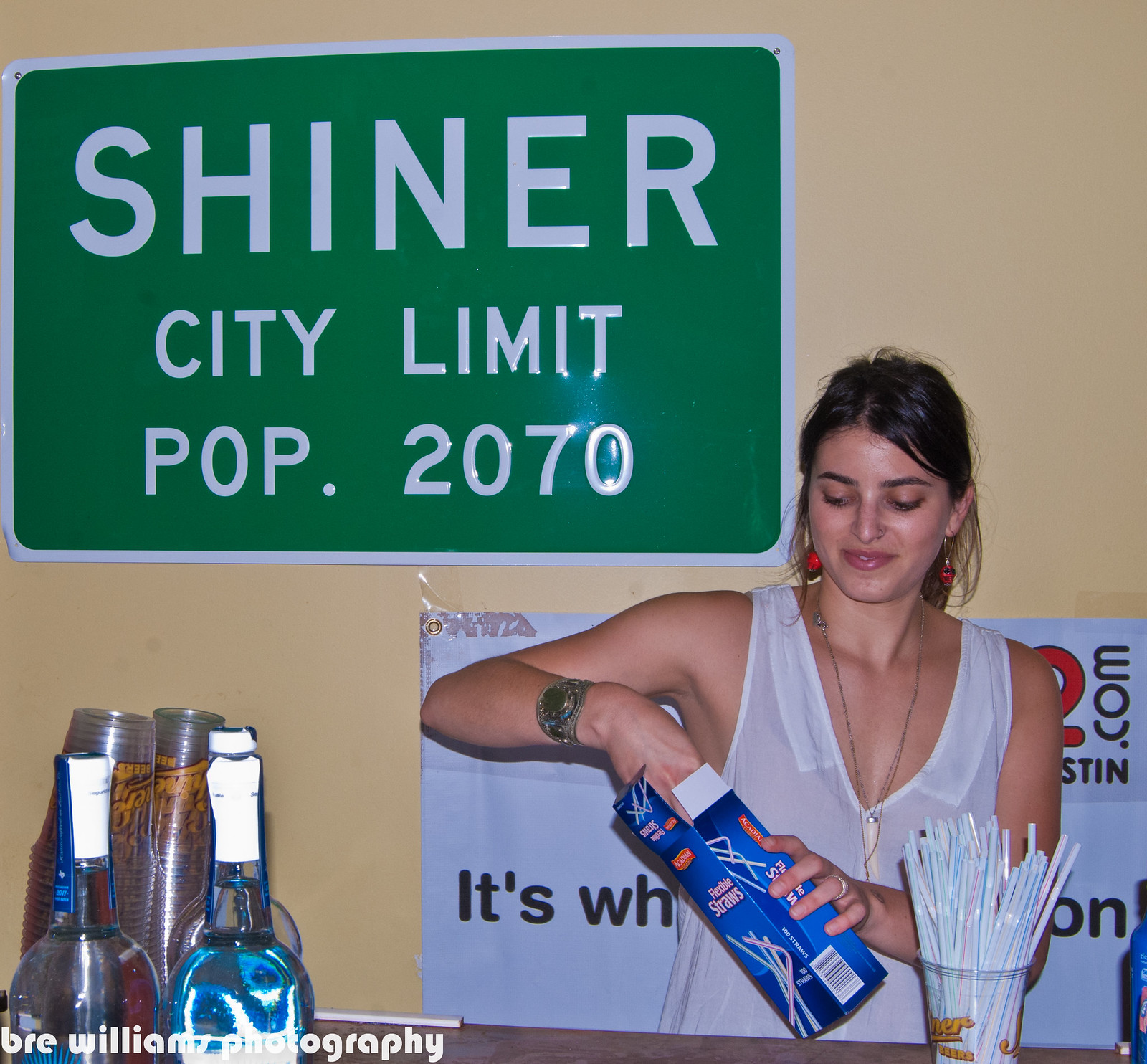The indoor photograph captures a medium-dark-skinned girl with dark brown, almost black hair, and dark features. She stands at a bar, dressed in a white, see-through blouse with red earrings and a chain around her neck. A watch adorns her right hand as she holds a blue box labeled "straws" and reaches inside it. In front of her, a glass already filled with white, blue, and red straws is visible next to two bottles and several empty plastic cups. Behind her on the wall is a street sign reading "Shiner City Limit POP 2070". The bottom portion of another sign can be seen, featuring only the word "It's". The left-hand corner of the photograph is marked with "Brie Williams Photography" in a computer-generated font, suggesting it could be an advertisement.